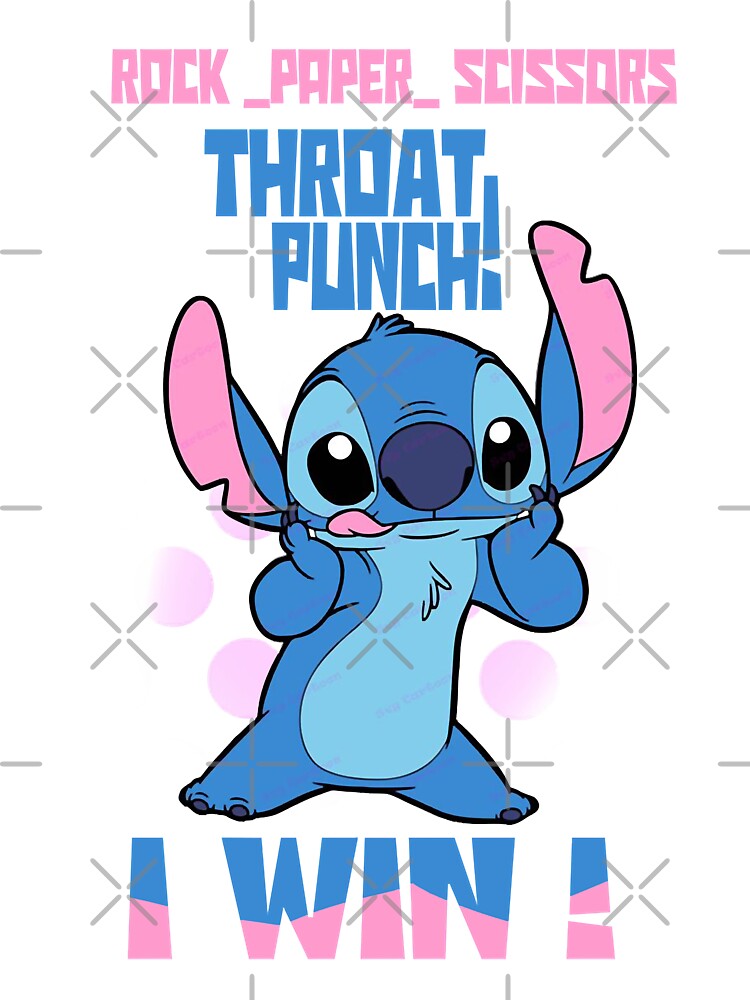The image is a computer-generated graphic featuring the Disney character Stitch from "Lilo and Stitch." Stitch is depicted in a medium shade of blue with lighter blue on his stomach and tufts of fur on his head and chest, as well as pink ears and tongue sticking out. His eyes are black and white, adding to his cute expression with his hands up to his face and feet stretched out. Text overlays the image in a vibrant combination of pink and blue fonts. At the very top, it reads "rock_paper_scissors" in pink, followed by "throat punch!" in blue. At the bottom of the image, the phrase "I win!" is displayed in both pink and blue. The background is white with scattered pink circles and numerous crosses, enhancing the playful and whimsical feel. The image itself is rectangular, with watermark-style designs hinting that it may be a SVG graphic design.